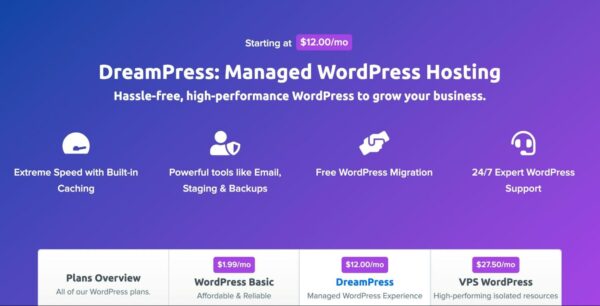The image depicts a screenshot of an advertisement positioned near the top center, promoting DreamPress managed WordPress hosting starting at $12 per month. The ad highlights the benefits of this hosting service, stating: "Hassle-free, high-performance WordPress to grow your business." Four icons are displayed, each representing key features:

1. "Extreme speed with built-in caching."
2. "Powerful tools like email, staging, and backups."
3. "Free WordPress migration."
4. "24/7 expert WordPress support."

Below the advertisement, part of a pricing chart is visible, though partially cut off, listing different WordPress hosting plans:

- **WordPress Basic**: Priced at $1.99 per month, offering affordable and reliable service.
- **DreamPress Managed WordPress**: Priced at $12 per month, referred to as the DreamPress managed WordPress experience.
- **VPS WordPress**: Priced at $27.50 per month, providing high-performing, isolated resources under this plan.

The chart header indicates an overview of all the WordPress plans available.